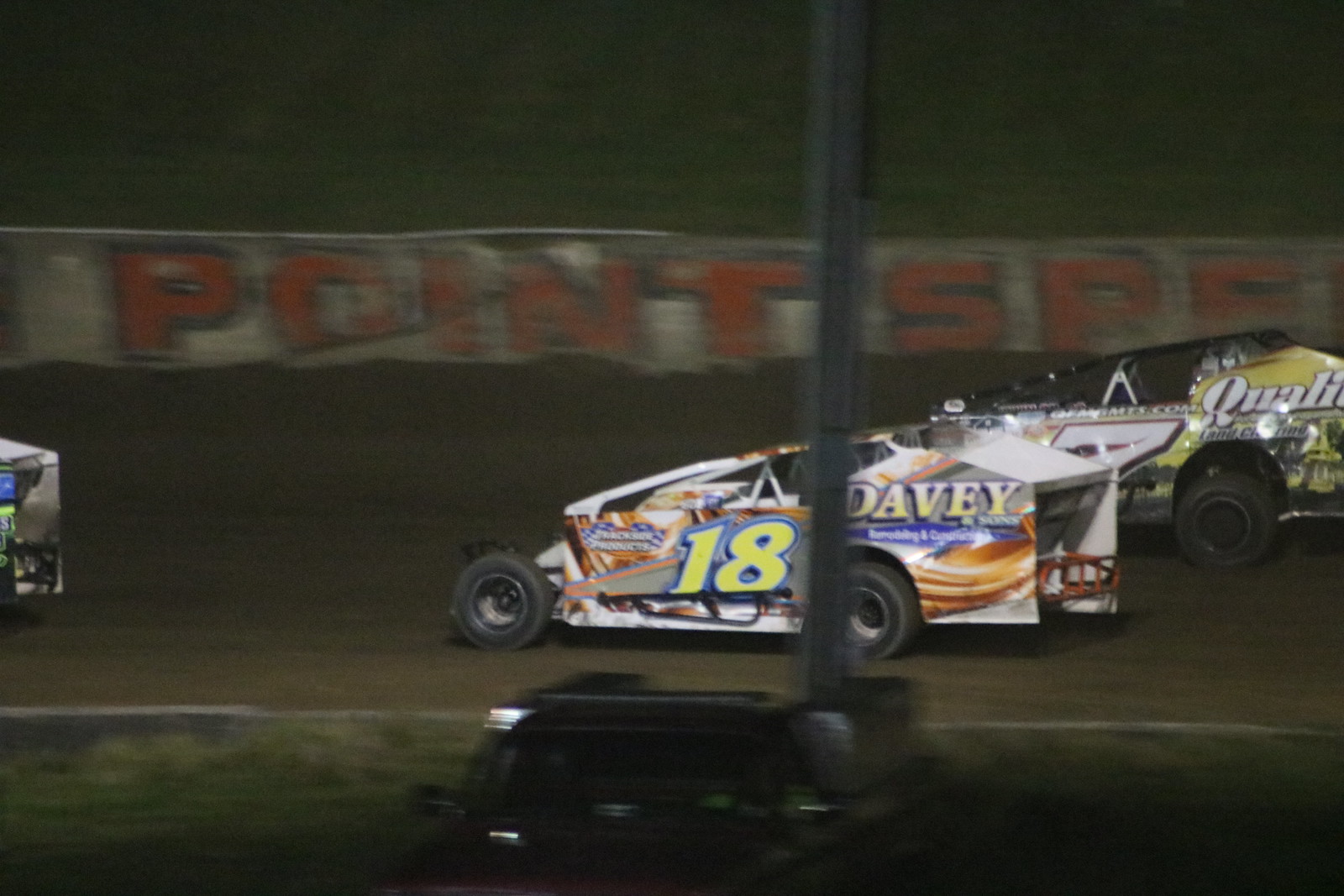This detailed color photograph captures a nighttime auto race on a dark brown dirt track bordered by white lines. At the center of the image is a white race car adorned with a brown and purple design, prominently displaying the number 18 in bold yellow surrounded by blue, along with the name "Davey" also in yellow on blue. The car races from left to right with black tires cutting through the dirt. In the background, partially obscured by a pole that extends out of the frame at the top, a white barrier with large orange letters reads "POINTSPE" and separates the track from a grassy area beyond. Another visible race car to the right, painted yellow with the word "Quality" in white text, shares the track. In the immediate foreground, a darker parked vehicle and grass can be seen on the right side, past the railing. The image captures the energy and vibrant colors of the race under night conditions, framed by the bustling details of the race track environment.